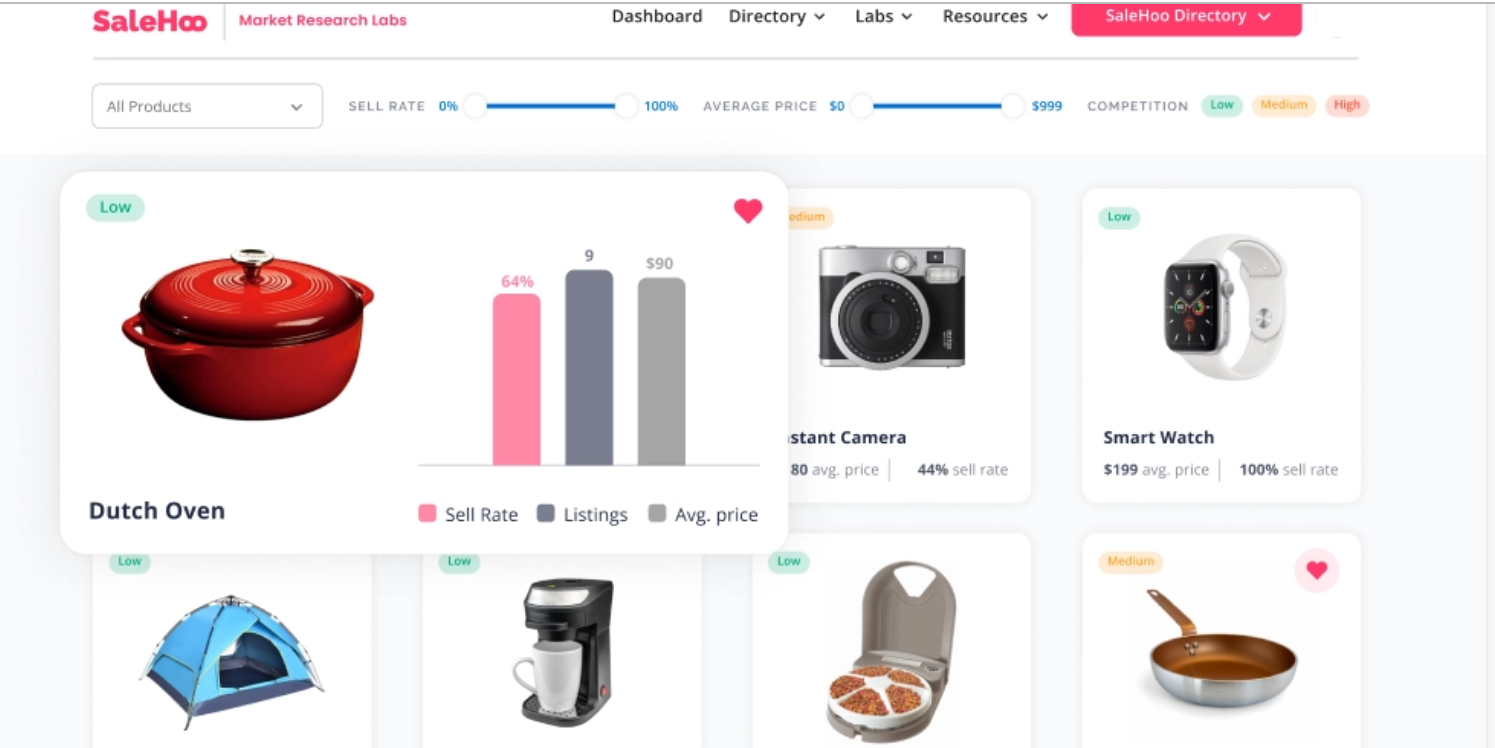The image features a predominantly white background, with the center and bottom sections showcasing a light gray rectangular box. In the top left corner, the word "SALE" is displayed in pink text, accompanied by slightly smaller pink text to the right that reads "Market Research Labs." Further to the right, three more headers appear in black text: "Dashboard," "Directory," "Labs," and "Resources," respectively. Adjacent to these headers, on the far right, there is a pink rounded rectangular box containing white text that reads "SALE WHO Directory."

Beneath the "SALE WHO" text in the top left, there is a white box with light gray text that says "All Products." Moving to the right of this, there are blue slider controls with circular white buttons for adjusting settings. Below these sliders, the image showcases various product images: 

1. On the top left, a red Dutch oven is prominently displayed.
2. To the right of the Dutch oven, there is a bar graph with pink, gray, and light gray bars, with the gray bar being the longest, followed by the light gray bar, and the pink bar being the shortest.
3. To the right of the bar graph, a black and silver camera is shown.
4. Next to the camera, there is a smart watch.
5. In the bottom left corner, a blue open tent is visible.
6. To the right of the tent, there is a coffee maker with a mug inside.
7. Adjacent to the coffee maker, there is a light gray container.
8. Finally, in the bottom right corner, a silver saucepan is displayed.

This detailed assortment of items, alongside various textual elements, provides a comprehensive view of the interface and its functionalities.